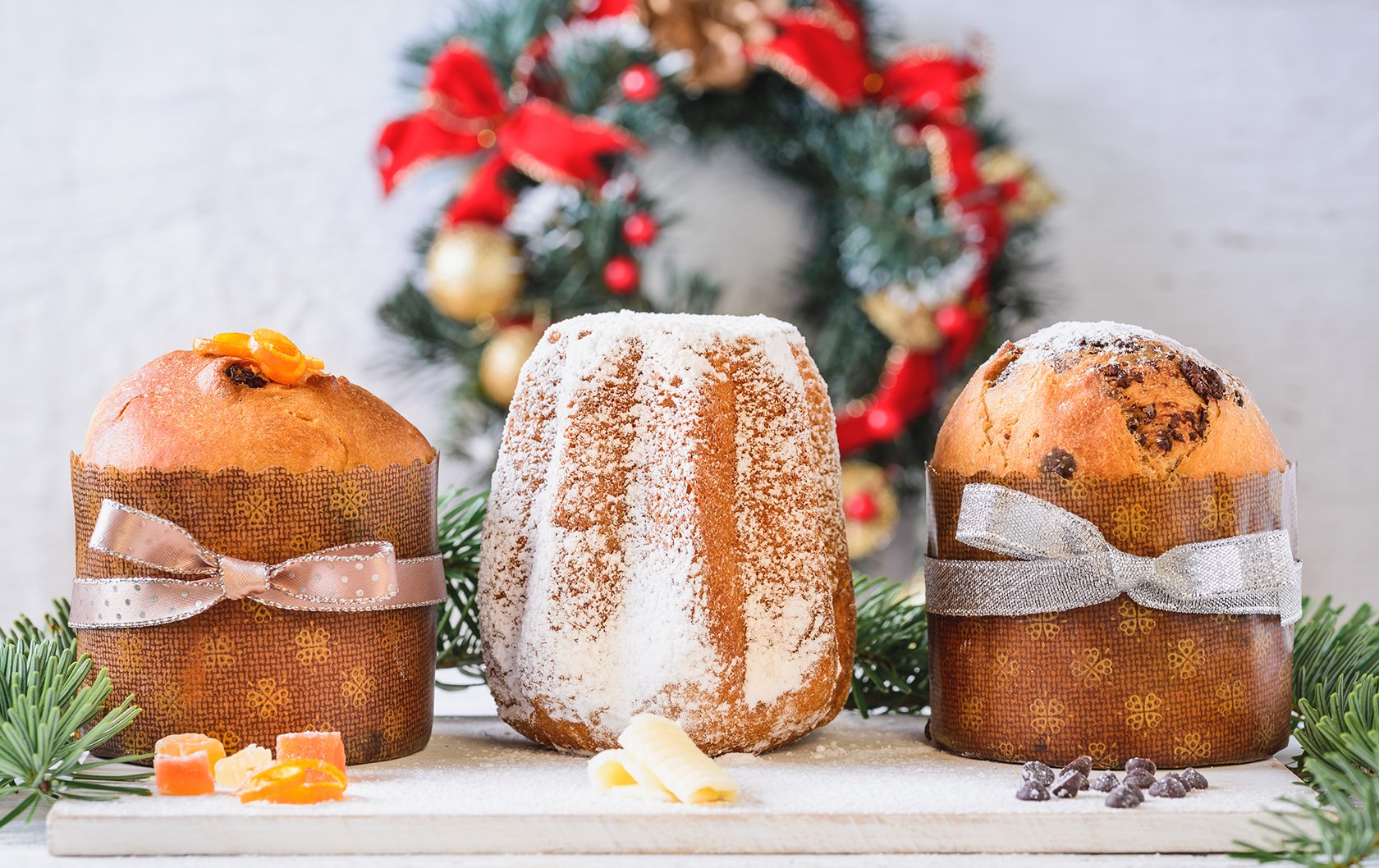This detailed photograph presents a festive Christmas display featuring three cylindrical pastries, prominently arranged on a white wooden cutting board. The left and right pastries are elegantly wrapped in flower-patterned parchment paper, secured with silver bows, and each exhibits unique garnishes. The left pastry is adorned with candied orange peels, while the right one features chocolate chips at its base. The central pastry, towering over the others, is dusted generously with powdered sugar. A blurry Christmas wreath decorates the background, adding to the holiday ambiance with its red ribbons, gold ornaments, and green pine needles. This composition evokes a warm, celebratory spirit, highlighting the festive bakery treats as the focal point amidst the seasonal decor.